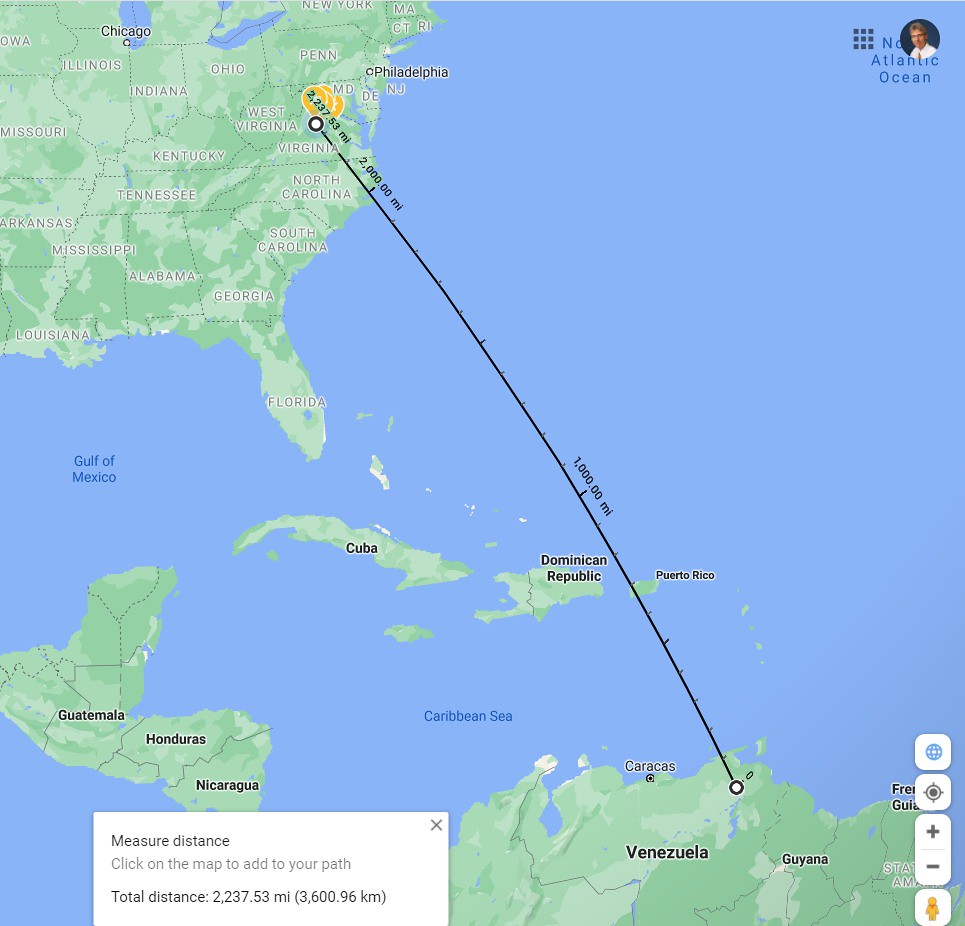This is a detailed screenshot of Google Earth focusing on the eastern United States. The map spans from parts of the Midwest, including states like Iowa, Missouri, and Arkansas, through to the eastern seaboard, highlighting states such as West Virginia and Virginia. Each state is labeled in black text with a white background. Over a blue water backdrop representing the Atlantic Ocean, a black line illustrates a distance measurement, stretching from an area between West Virginia and Virginia down to Venezuela, covering a total distance of 2,237.53 miles. Along this path, the distance is marked at intervals of 1,000 and 2,000 miles. Notable locations include Puerto Rico, the Dominican Republic, Cuba, Guatemala, Honduras, and Nicaragua. The map features a legend in the bottom left corner, which provides measurement instructions, stating to "click on the map to add to your path." The visual includes orange circles along the black line, indicating key points. In the top right corner, a small white circle contains the image of a person with brown hair, light skin, wearing black glasses, a white collared shirt, and a brown tie, placed above the North Atlantic Ocean. The map employs different shades of green, with a lighter sage and darker sage denoting various geographical regions.